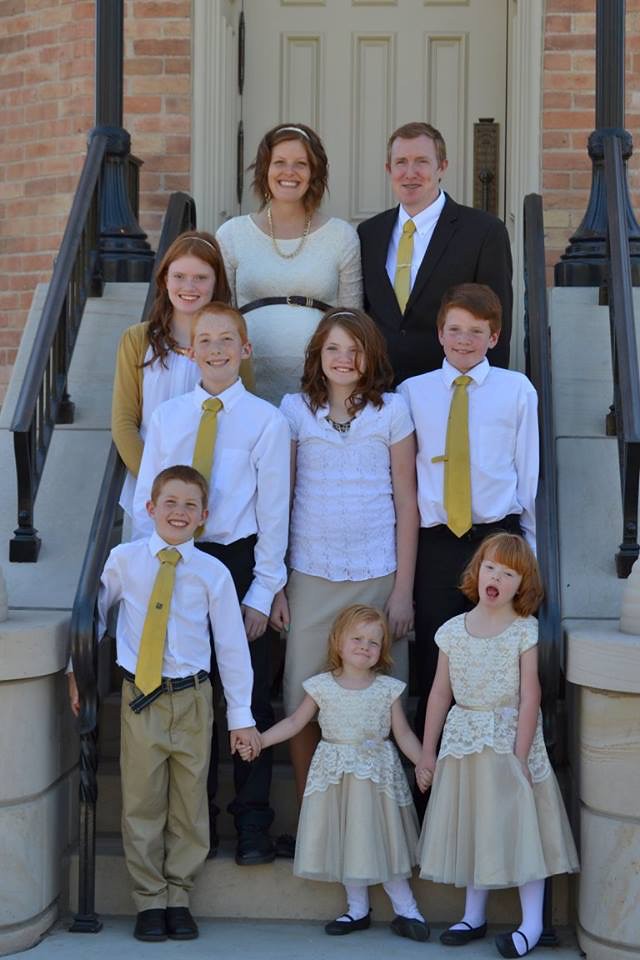This outdoor family photograph captures a joyful family of nine standing closely together on a brick church's concrete staircase, framed by black iron rails. At the top left stands the smiling mother, dressed in a tan dress with short hair, right beside her is the father, wearing a black suit with a matching yellow tie. Below them, their seven children are neatly arranged in three descending rows. The older girl in the second row center wears a yellow cardigan over her white shirt and brown skirt. Flanking her are two older boys in white button-up shirts, yellow ties, and black pants. On the bottom row, three boys and four girls are arranged symmetrically. All boys don white shirts with yellow ties, with the youngest boy in khaki pants. The littlest girls and the girl next center front wear matching beige lace dresses with black shoes. The entire family shares distinctive reddish-brown hair, adding a cohesive charm to the scene. The children are all smiles, radiating happiness, while everyone seems coordinated and harmonious in their attire.